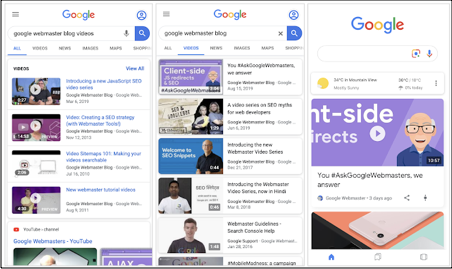The image presents a side-by-side comparison of three mobile screenshots showcasing different Google search results and content. Due to the low resolution, some of the text is not fully legible, but key details can be discerned:

- The left screenshot highlights the search term "Google Webmaster blog videos." Below the search bar are several video thumbnails. The first video appears to introduce a new video series, followed by videos on creating an SEO strategy, making videos searchable, and new webmaster tutorial videos.

- The middle screenshot shows a search for "Google Webmaster blog." It lists videos covering topics such as SEO myths for web developers, answers about Google Webmasters, an introduction to the new webmaster video series, webmaster guidelines, and Search Console help.

- The right screenshot is more distinct in its content, featuring prominently two videos. The top video, set against a purple background, is an animated clip showing an elderly man in glasses wearing a blue shirt, smiling. The text nearby includes hashtags such as "#YouAsk" and "#AskGoogleWebmasters," suggesting an interactive or Q&A format. The bottom of this screenshot depicts an image of a phone on a pink desk.

Additionally, the weather icon indicates that it is a sunny day, with a clear depiction of the sun. This detail subtly adds to the context of the mobile environment in which these screenshots were taken.